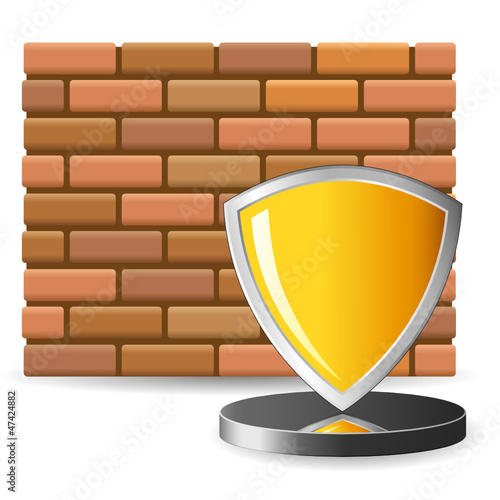The image is a graphic, not a photograph, depicting a surreal and slightly perplexing scene. The background features a brick wall composed of alternating rows of bricks in shades of brown-orange, yellow-orange, and various shades of brown, with brown grout in between. There are nine rows in total. Printed diagonally across the bricks is the watermark, "Adobe Stock." 

In the foreground, slightly to the right, there's an abstract, upside-down triangular shield with a silver border. The shield itself is a gradient yellow, transitioning from light to dark from left to right, and it features a white reflective gleam on its surface. This shield appears to defy gravity, balancing delicately on its point atop a reflective, silver-gray platter, which, in turn, sits on a white surface. The bottom of the shield is mirrored in the shiny platter, adding to the graphic's surreal quality.

In the bottom left corner of the image, the text "Adobe Stock" can be seen running vertically, along with the stock number 47442882. This caption underscores the fact that the image is a stock graphic available from Adobe Stock.